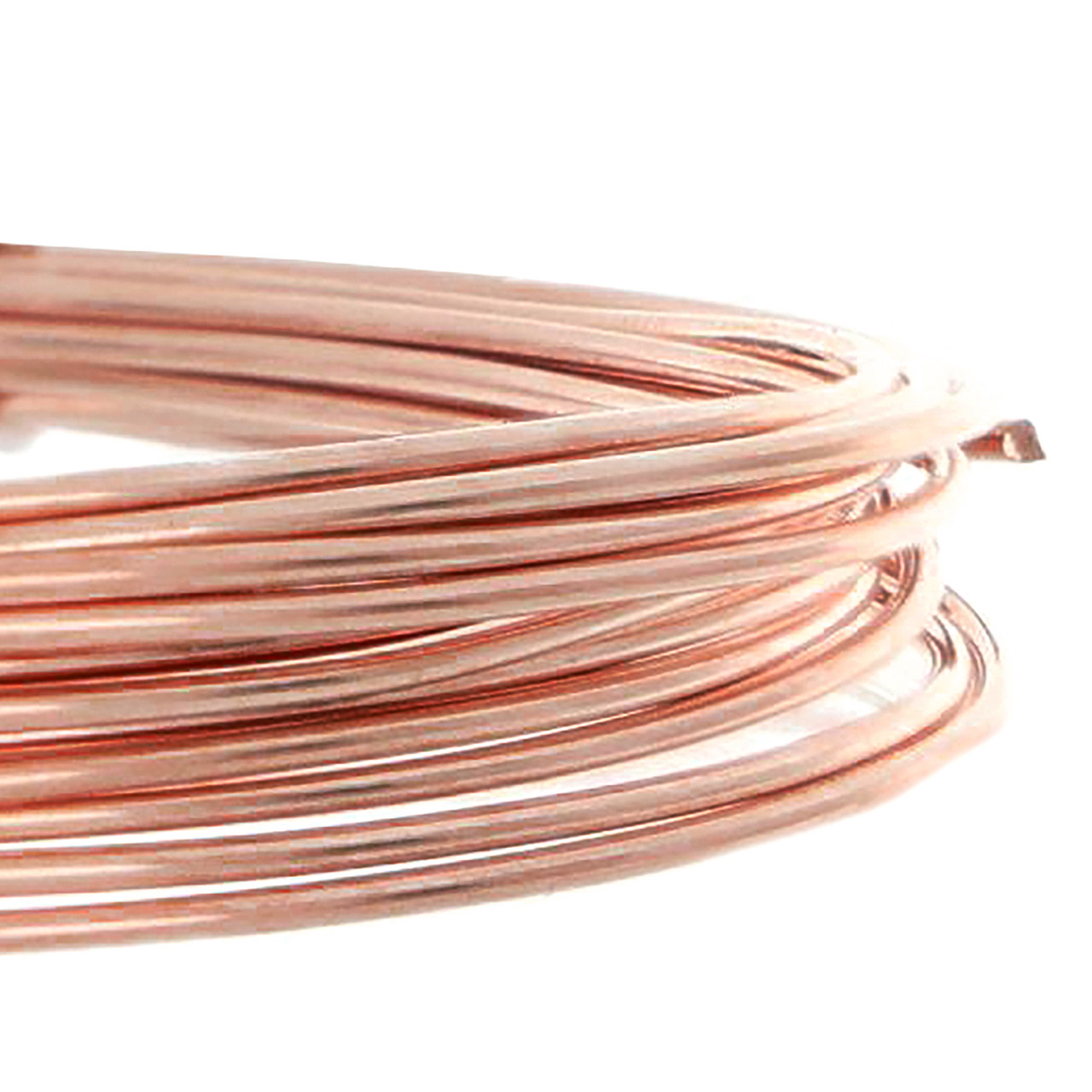This photograph features a neatly wound, shiny copper tubing coiled into approximately ten to twelve loops. The tubing has a light orange, almost pristine appearance, indicating minimal exposure to air and oxidation. The image captures about one-third of the coil, occupying the center right of the frame. The background is plain white, making the copper tubing stand out with little to no shadows. The copper wiring is relatively thick, roughly the width of a finger, and although cropped, it is evident that it is meticulously wound. The overall composition is simple yet detailed, emphasizing the clean, orderly arrangement of the copper coils.